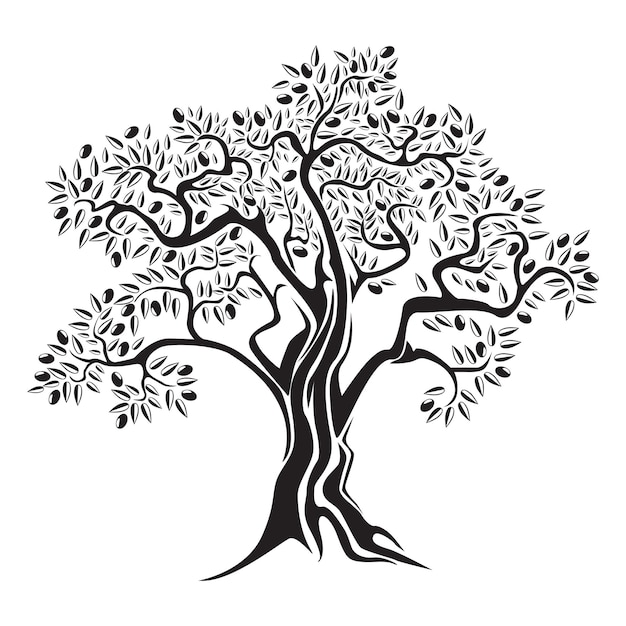The image displays a minimalistic and stylized drawing of a deciduous tree rendered entirely in black on a white background. The tree features a large trunk with roots anchoring it, and from the top, multiple major branches jut upward in various directions, such as up and slightly to the left, right, or center. These branches hold numerous smaller offshoots adorned with an abundance of leaves. The leaves are minimalist in design, split vertically with one half black and the other white, giving a striking contrast. Each leaf varies in shape, including circular, oval, and pear-like forms, and they are oriented in multiple directions contributing to a sense of natural authenticity. No color is used in the drawing apart from black, with details filled in by the white negative space, which creates a somewhat see-through effect. The lack of any other elements emphasizes the solitary presence of the tree, with its intricate branches and detailed leaves.